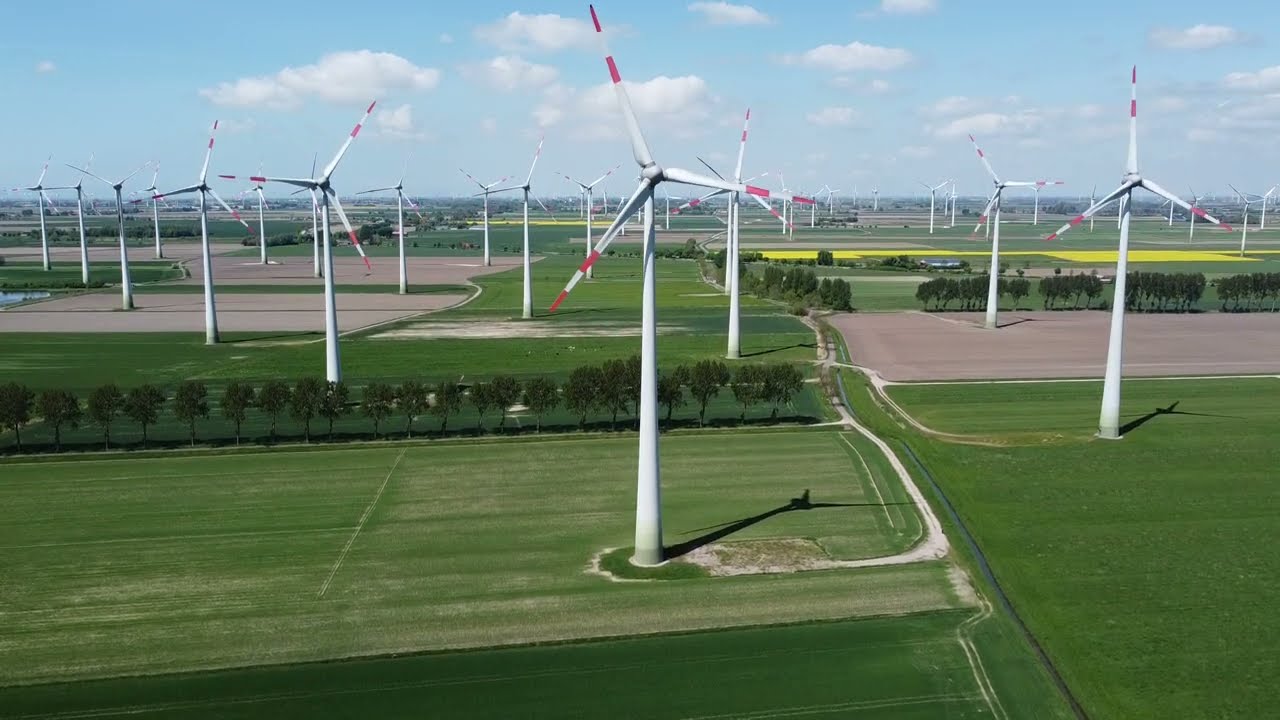In this vivid aerial image, we observe a sprawling windmill farm set within expansive, open farmland. The farm features numerous modern wind turbines with light gray metal bases and large three-bladed propellers that are predominantly white with red tips. The central focus is a prominent windmill, situated in the middle of the frame, with approximately twenty additional windmills receding into the distance.

The landscape is a patchwork of agricultural fields in varied hues, ranging from vibrant greens and yellows to light tans. These fields are interspersed with tree lines of small green-leaved trees, dividing the crop areas. The terrain includes both stretches of green grass and sections of light brown dirt or concrete where some windmills are anchored.

Above this picturesque scene, a bright blue sky is adorned with puffy white clouds, suggesting a clear, sunny day. The perspective, possibly from the top of a tall building or an aerial vantage, aligns with the height of the windmills, offering an expansive view without any textual elements disrupting the natural scenery.